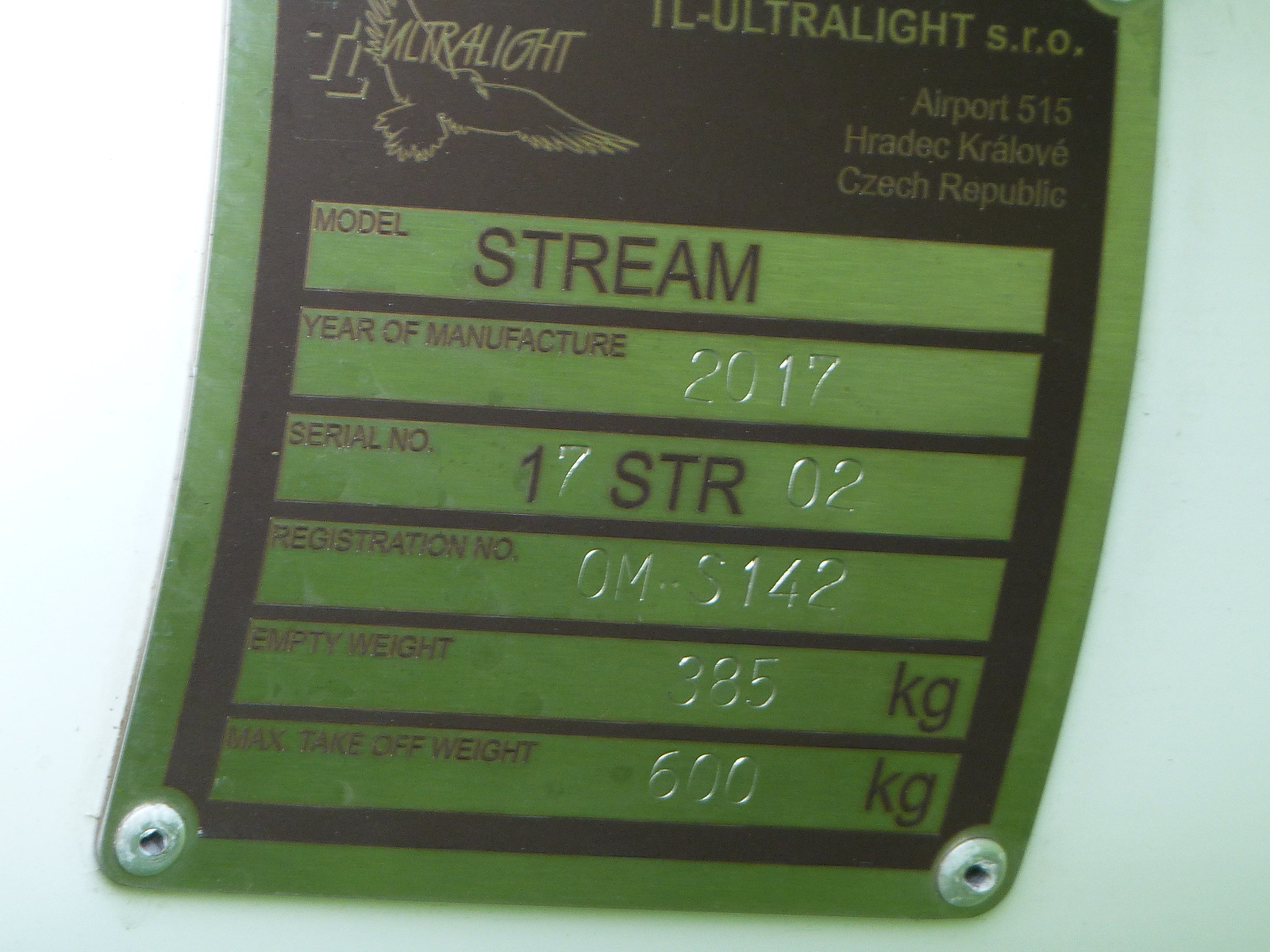The image depicts a durable green metal label, firmly bolted with steel rivets onto an unidentified structure, likely an aircraft. The label displays various technical details pertinent to the object it is attached to. At the very top on a black background with green lettering, the label reads "ULTRALIGHT AIRPORT 515, HRADEC, CZECH REPUBLIC." The upper left corner features an image of an eagle next to the word "ULTRALIGHT TL." Central to the label, in capital black letters, is the model name "STREAM," alongside the year of manufacture, 2017. Also engraved are essential specifications: serial number 17STR02, registration number 0MS142, empty weight of 385 kilograms, and a maximum takeoff weight of 600 kilograms. The background color of the structure holding the label appears to be light blue or white, adding contrast and making the label more readable.